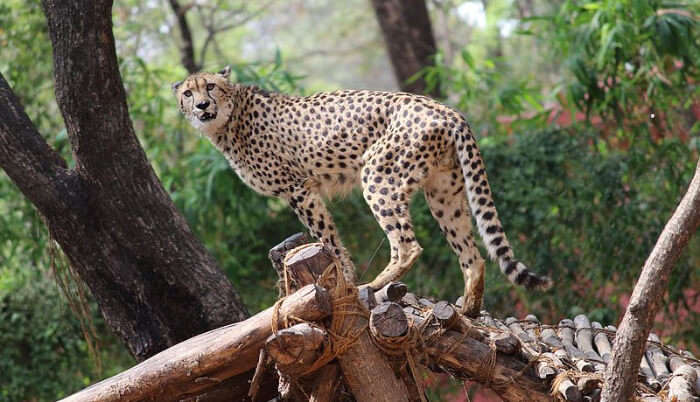The photograph captures a majestic cheetah in a zoo, poised atop a primitive, man-made wooden structure, which resembles a rudimentary bridge or platform composed of logs tied together with twine. The cheetah, instantly recognizable by its light tan fur and distinctive black spots, stands with its sleek, muscular body facing left, while its head is turned towards the camera, locking eyes with the viewer. Its elongated tail curves gracefully as it rests. In the backdrop, a lush forested area with abundant green leaves and prominent tree trunks creates a naturalistic setting, though the gray, washed-out sky hints at overcast conditions. The composition is completed by the presence of a massive tree trunk branching into a V-shape and a variety of low bushes, all contributing to the wild yet curated ambiance of the zoo environment.